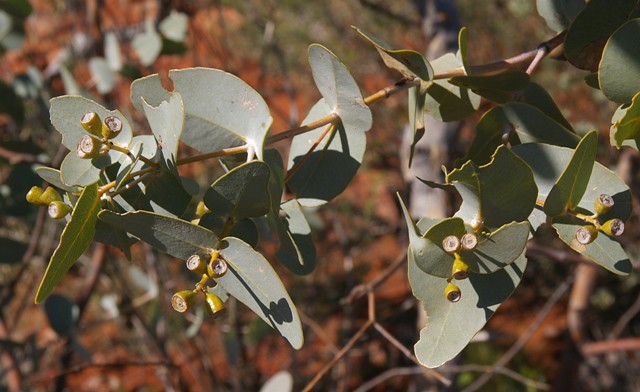This outdoor photograph, taken in bright sunlight, showcases a close-up view of a bent green stem entering from the upper right and stretching horizontally to the left. Broad green leaves, showing noticeable signs of insect damage likely caused by caterpillars, are attached at various points along the stem. The leaves display a striking contrast with a darker and a paler side. The stem is adorned with round, conical buds that are green on the outside and light white on the inside, resembling bell or cup shapes that may blossom later. The background of the image is a blurred mix of sunlit tree leaves, twigs, and earthy tones with hints of fall colors, emphasizing the wild and natural setting. There is no text or print on the image.